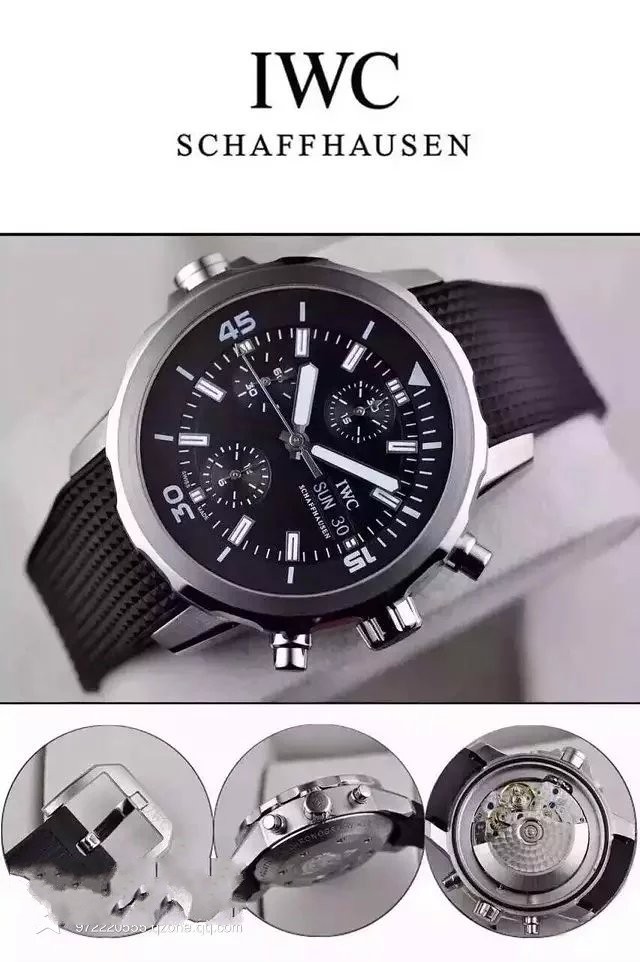This vertical image is a sophisticated advertisement for the renowned watch brand, IWC Schaffhausen. The top section features a minimalist design with black, all-caps serif text on a white background, confidently displaying "IWC" followed by "Schaffhausen" below it. Centered in the middle of the image is a high-resolution photograph of a luxurious watch, showcasing its elegant black band, polished silver frame, and intricate black watch face. The face is adorned with a myriad of technical details, including multiple smaller dials and a dedicated date section, emphasizing the watch’s functionality and precision. Along the bottom of the image, three small, circular insets provide close-up views of the watch's exquisite craftsmanship. One circle highlights the refined clasp, another focuses on the detailed side profile with its crown, and the third reveals the intricate inner mechanisms and underside of the watch, showcasing the brand's commitment to high-quality engineering and design. This compelling visual compilation effectively conveys the sophistication and technical prowess of IWC Schaffhausen timepieces.